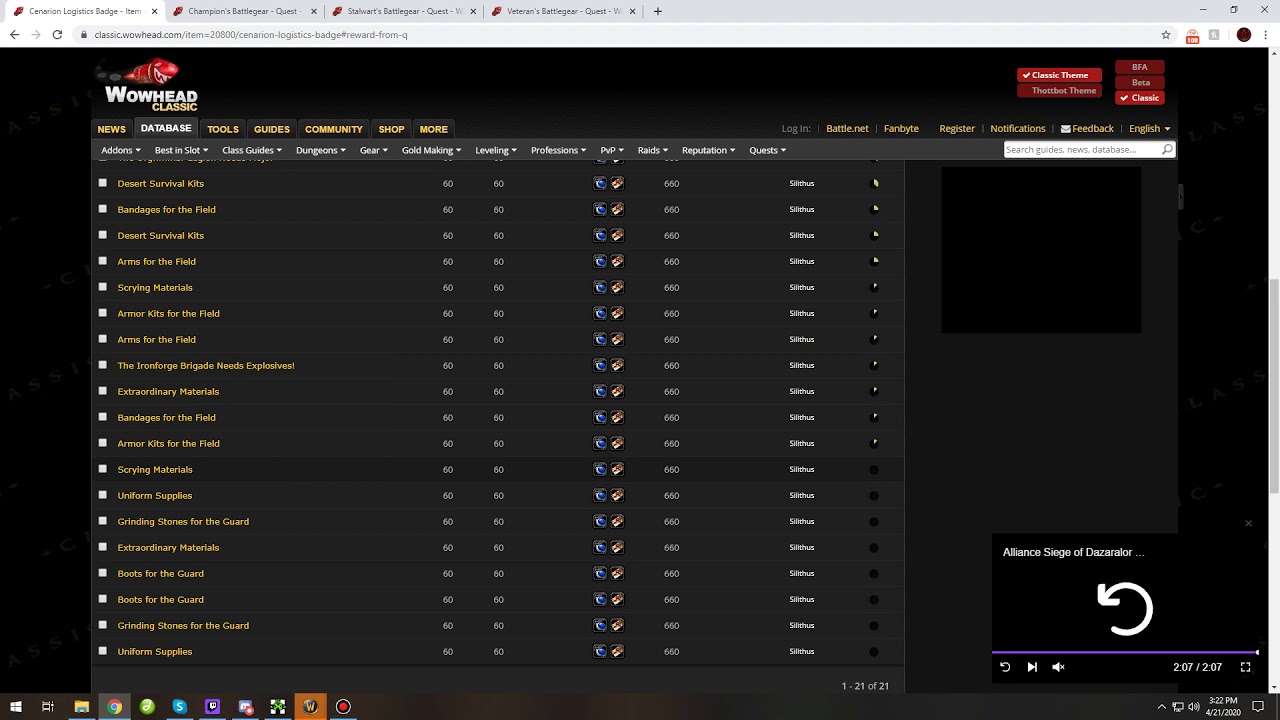Screenshot of the Wowhead Classic website displaying multiple open tabs with various item lists. The interface shows a detailed array of inventory items and categories, including "Scenario Logistics Badge," "Champion's Battle Gear," "Stalwart's Battle Gear," and "Veteran's Battle Gear." The top-left corner prominently features the Wowhead Classic logo. Navigation options such as "News," "Database," "Tools," "Guides," "Community," "Shop," and "More" are clearly visible. Specific item categories detailed include "Desert Survival Kits," "Bandages for the Field," "Arms for the Field," "Scrying Materials," and "Armor Kits for the Field." The interface also lists various in-game needs like "The Ironforge Brigade Needs Explosives," "Uniform Supplies," "Grinding Stones for the Guard," and "Boots for the Guard." A tab labeled "Items" suggests a focus on item retrieval or inventory management. Additional options at the bottom indicate filter categories like "Add-ons," "Best-in-Slot," "Guides," "Dungeons," "Gear," "Gold Making," "Leveling," "Professions," "PvP," "Raids," "Reputation," and "Quests." The website's theme can be customized with options for Classic, Thoughtbot theme, BFA, and Beta Classic. A Twitch mini-player appears minimized in the bottom-right corner, offering a holistic, interactive experience for World of Warcraft players seeking in-depth information on gear and quests.